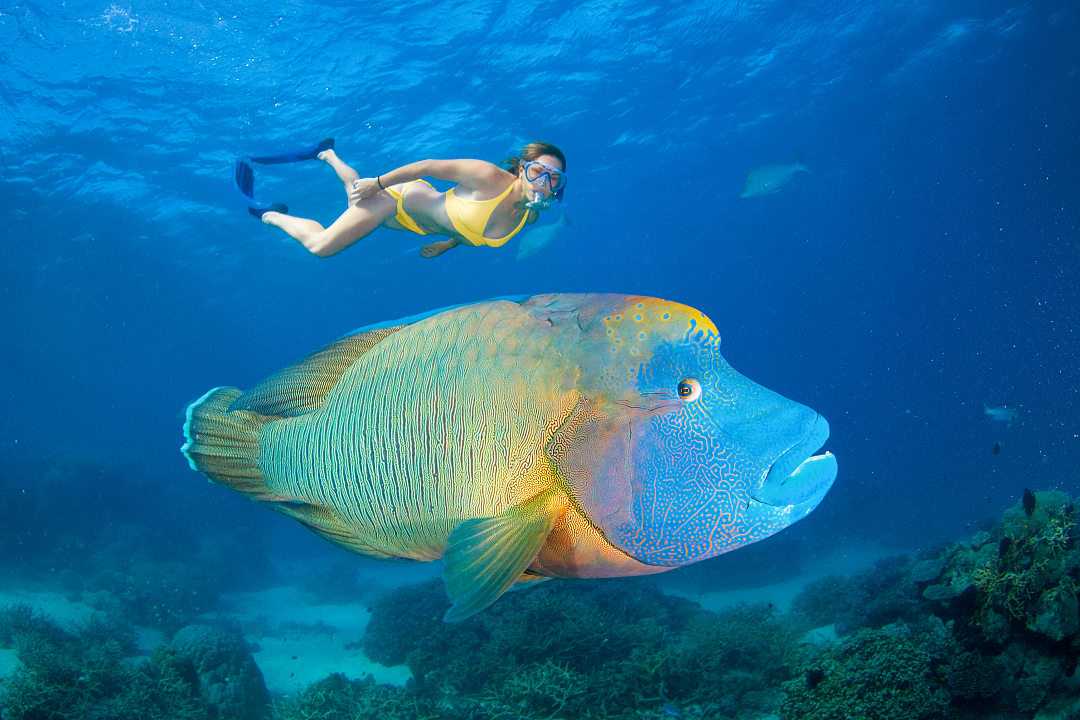In a vivid underwater scene with a bluish tint, a photograph captures a mesmerizing encounter between a snorkeler and a colossal, vibrantly colored fish. Set against a backdrop that transitions from a lighter blue near the forefront to a deep blue void in the distance, the rectangular image showcases intriguing marine life. The center of the photograph features an enormous fish with a unique palette of colors: a blue head adorned with intricate yellow lines, large white and black eyes, and prominent blue lips framing its partially open mouth. Its scales are a striking mix of yellow, blue, and hints of green, with distinctive markings like a white stripe on the tail fin edge and a black stripe on the back fin.

Hovering gracefully above the fish is a woman in a yellow two-piece swimsuit, sporting blue swim fins, a blue-framed set of goggles, and a white snorkel. Her brown hair flows freely in the water as she enjoys her underwater adventure. The clarity of the water reveals additional details: light brown sand, patches of green sea vegetation, and scattered earthy colored rocks on the sea floor. The image, possibly taken in a tropical locale, skillfully blends elements of the natural underwater environment with the striking presence of the fish and the snorkeling woman, creating a captivating and immersive visual narrative.